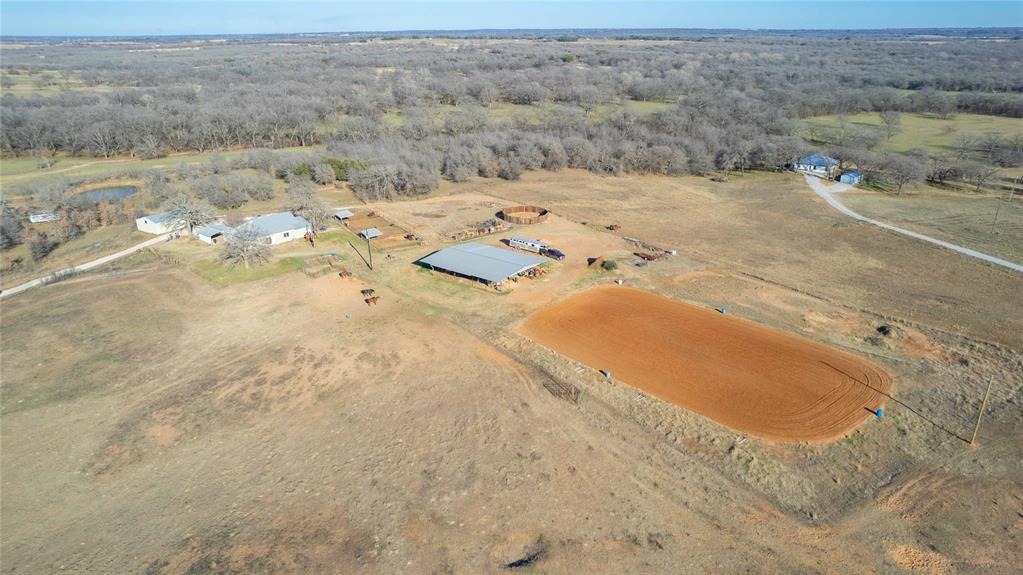This aerial photograph captures a stark, rural landscape under a clear blue sky. Dominated by dry, barren land with sparse vegetation, the scene features several white, single-story dwellings with dark, possibly green roofs. Toward the top of the image, a grove of gray, lifeless trees lines the horizon, suggesting prolonged dry conditions. In the lower section, there is an oval patch of smoothed dirt, differing in color from the surrounding area, hinting at recent preparation—perhaps for livestock or construction. Scattered throughout the image are a few small animals, likely cows or horses, grazing on the sparse, dry ground. On the left side, a small pond near one of the houses provides a rare touch of water amidst the arid environment. Roads weave through the landscape, connecting houses and leading to various structures, including what appears to be an open-air area that could potentially serve as a chicken coop. The overall impression is one of a remote, farm-like area struggling against the harsh conditions of a parched land.